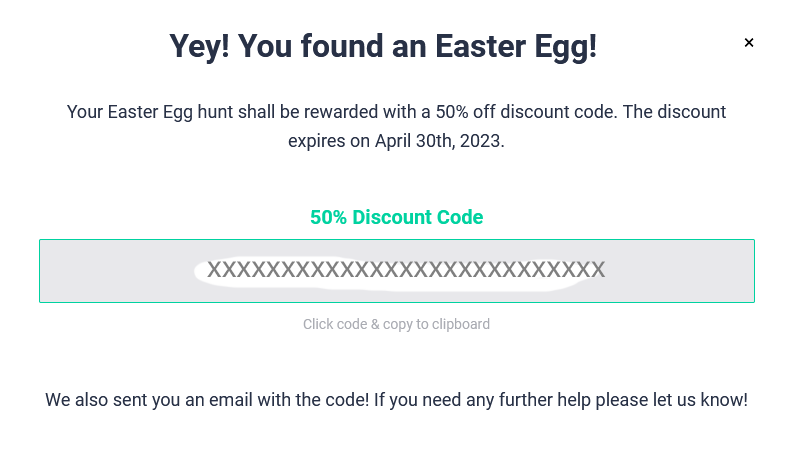The image is a screenshot of a pop-up box from a website, displayed against an all-white background. At the top of the pop-up, bold black letters announce, "Yay! YaY! You found an Easter egg!" Below this message, the text explains, "Your Easter egg hunt shall be rewarded with a 50% off discount code. The discount expires on August 30th, 2023."

Further down, in a vibrant neon teal color, the text reads "50% discount code". The actual discount code, however, has been crossed out by the person who took the screenshot. They used white to obscure the code and replaced it with a string of uppercase "X" characters extending across the entire length of where the code would have been.

Below the modification, gray text instructs, "Click code and copy to clipboard." At the bottom of the pop-up, in black text, it states, "We also sent you an email with the code. If you need any further help, please let us know."